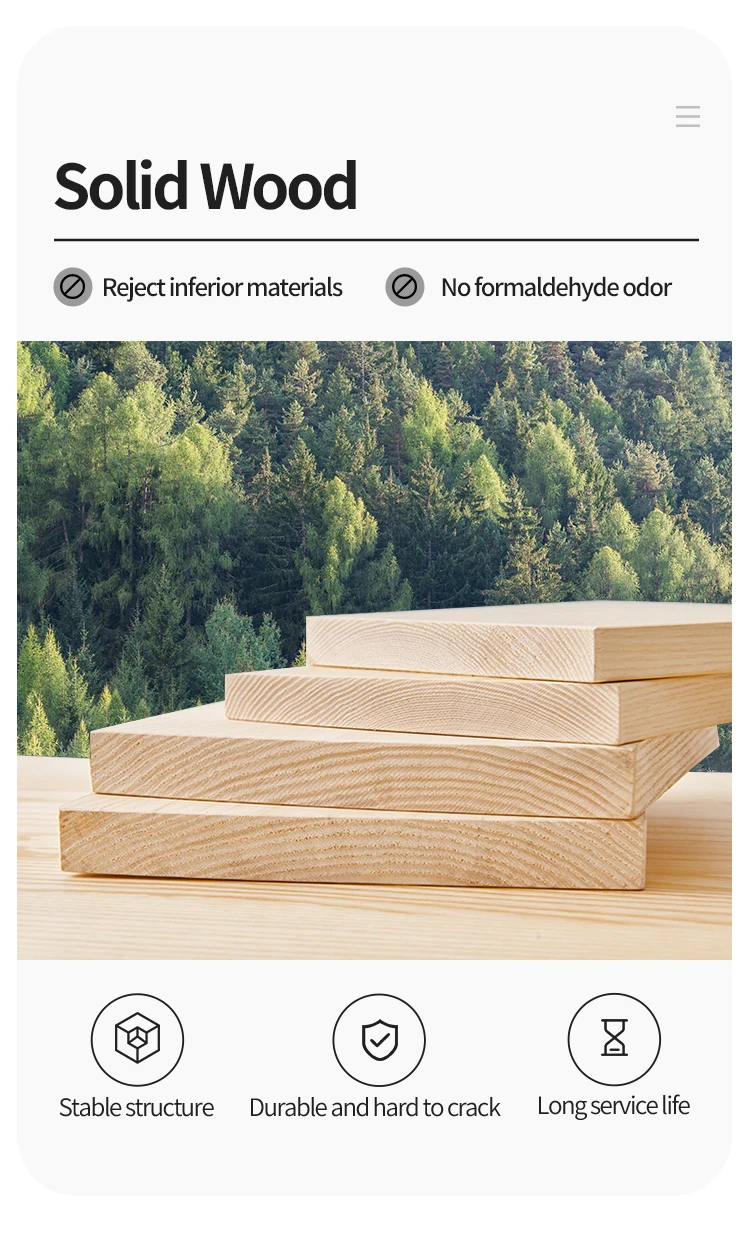Here is a detailed and cleaned-up caption for the described image:

---

Screenshot of a mobile-oriented webpage or app, featuring a background mostly shaded in off-white. At the top right corner, three horizontal lines suggest a drop-down menu. The top-left section displays the text "Solid Wood" in black font, underlined by a horizontal black line. Below, there's a "no symbol" (a circle with a diagonal line through it) outlined in gray, accompanied by the text "Reject Inferior Materials" inside the circle. Adjacent to it, another bullet point with a similar icon emphasizes "No Formaldehyde Odor."

The central portion showcases several fresh-cut, unstained 2x4 wooden planks arranged on a tabletop, also made of similar fresh-cut, unstained wood. The background presents a lush forest full of trees, hinting at the natural source of the wood. At the bottom of the image, three icons are aligned horizontally. The first icon is labeled "Stable Structure," the second "Durable and Hard to Crack," and the third "Long Service Life."

---

This caption provides a thorough and organized description that captures all the key details from the image.